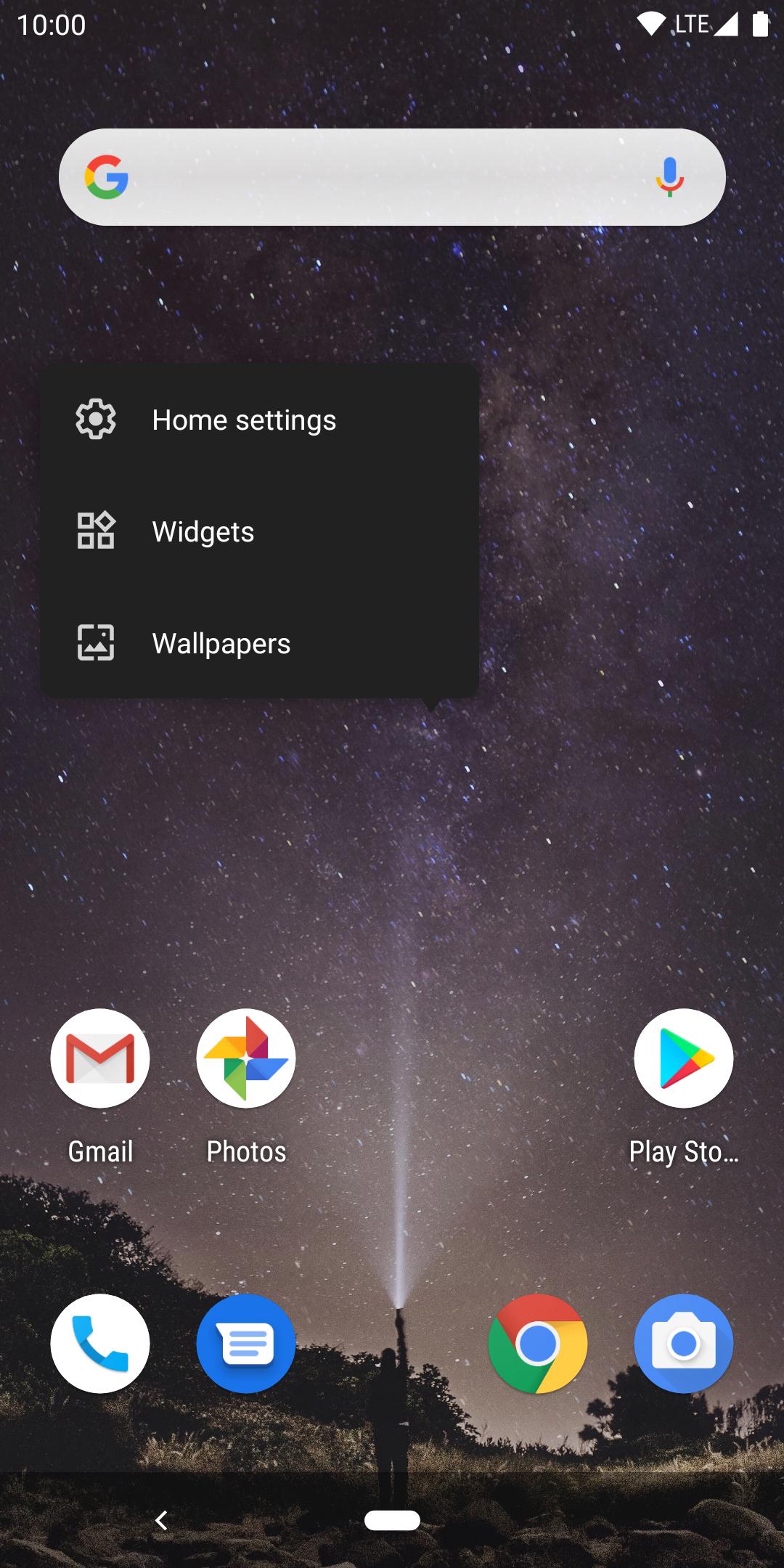The image is a screenshot taken on a smartphone with a backdrop depicting a serene starry night sky. Numerous stars are scattered across the night sky, creating a tranquil, cosmic atmosphere. At the bottom of the image, the silhouettes of trees and grass are visible, contributing to the natural setting. Within these silhouettes, a man is holding a flashlight, his right arm extended as he points the beam up towards the sky.

In the top left corner of the screen, the time is displayed in white text as "10:00". Nearby, on the right-hand side, icons for Wi-Fi strength, LTE connectivity, mobile service signal, and battery level are also in white.

Below this status bar, a white search bar is prominently featured. On the left of this bar is the colorful Google logo, with its capital 'G' rendered in red, yellow, green, and blue. At the right end of the search bar is a multicolored microphone icon - blue on top, yellow and red in the middle, and green on the bottom.

Beneath the search bar is a black navigation bar. On the left side of this bar is a white gear icon, labeled "Home settings". Next to it, an icon resembling a box composed of four smaller boxes is labeled "Widgets". To its right, an outline of a white box with two white mountains inside represents the "Wallpapers" function.

Within this section are several app shortcuts:
- A white circle with a red 'M', labeled "Gmail".
- A white circle with a fan-shaped symbol in yellow, green, blue, and red, labeled "Photos".
- Another white circle containing a blue phone icon.
- A blue circle with a white document icon, featuring three blue lines.
- A white circle with a multicolored play symbol (blue, green, red, yellow), labeled "Play Store".
- A multicolored circular ball with blue in the center, red on top, green on the left, and yellow on the right.
- A blue circle with a white camera icon.